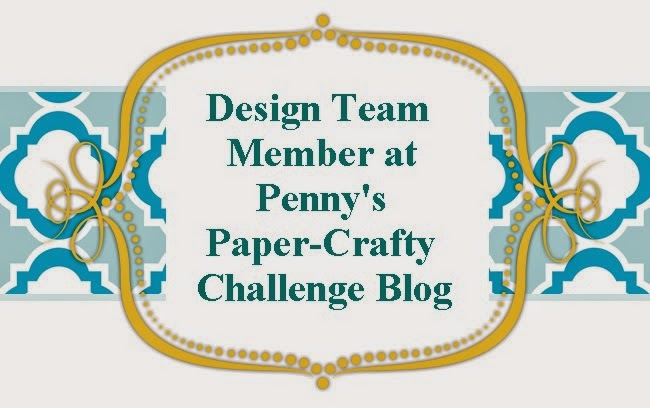The image showcases an elegant and meticulously designed banner, likely intended for a website or blog related to paper crafts. It features a light gray background adorned with sophisticated medium and light blue decorative elements and borders. On both the left and right sides, there are prominent, decorative rounded rectangle patterns in a yellow-gold hue, resembling ribbons adorned with bead-like details. These patterns frame a text area, where the words "Design Team Member at Penny's Paper Crafty Challenge Blog" are prominently displayed in dark gray-blue font. The overall aesthetic includes a harmonious blend of blue, light blue, white, and gold colors. The central text is positioned within a geometric pattern that evokes the design of an ornate tray or possibly a rug, enhancing the graphic's refined and stylish appearance. The entire composition has the air of a presentation slide or a sophisticated blog banner, emphasizing the artistic and design-focused nature of the content.